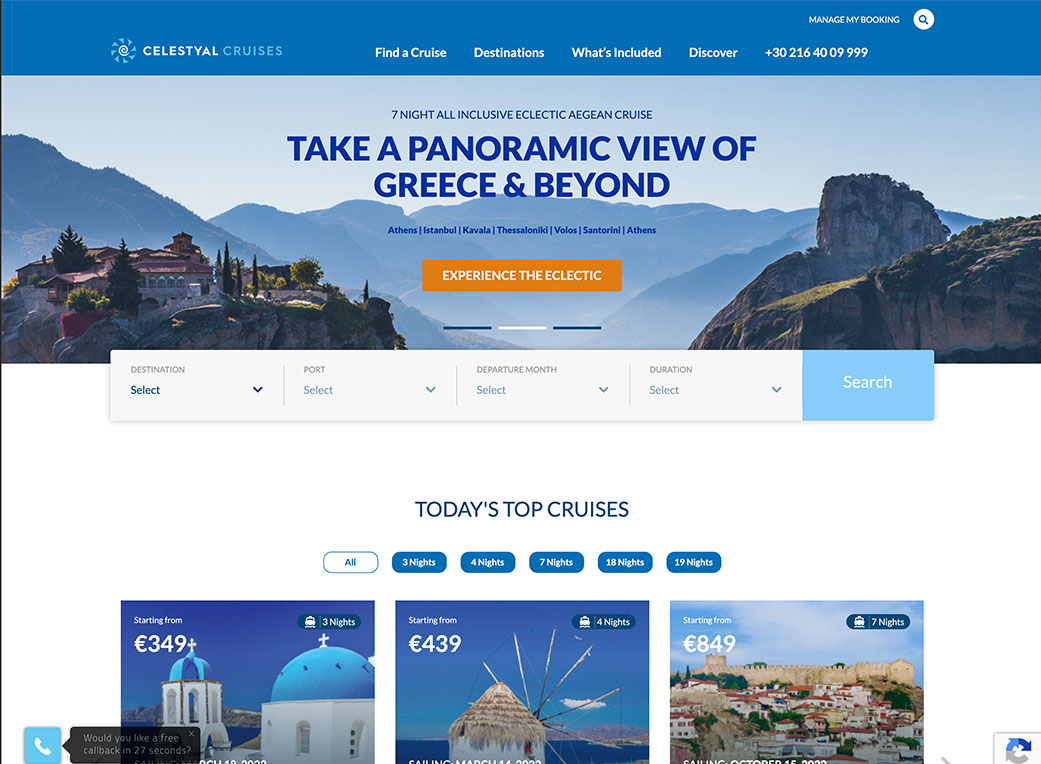The webpage for "Celestial Cruises" (spelled with a 'Y') features a prominent blue banner at the top. On the top left is the Celestial Cruises logo, and on the right, text noting that the service is "Managed by Booking" with a small hourglass icon next to it. Below this, there is a navigation menu with options for "Find a Cruise," "Destination," "What's Included," "Discover," and a contact phone number: +302164009999.

Highlighted on the page is an advertisement for a "Seven-Night All-Inclusive Eclectic Aegean Cruise," accompanied by a large, picturesque landscape photograph. This cruise offers a panoramic tour of Greece and beyond, including stops in Athens, Istanbul, Kavala, Thessalonica, Volos, and Santorini, before returning to Athens. There is an orange button with white text beneath the photograph that prompts visitors to "Experience the Eclectic."

Directly below this feature, there is a selection menu allowing users to customize their search for a cruise. Options include drop-down menus for choosing a destination (with the default being "Airport"), a departure month, the duration of the trip, and other preferences. A large search button is located on the right side of this section.